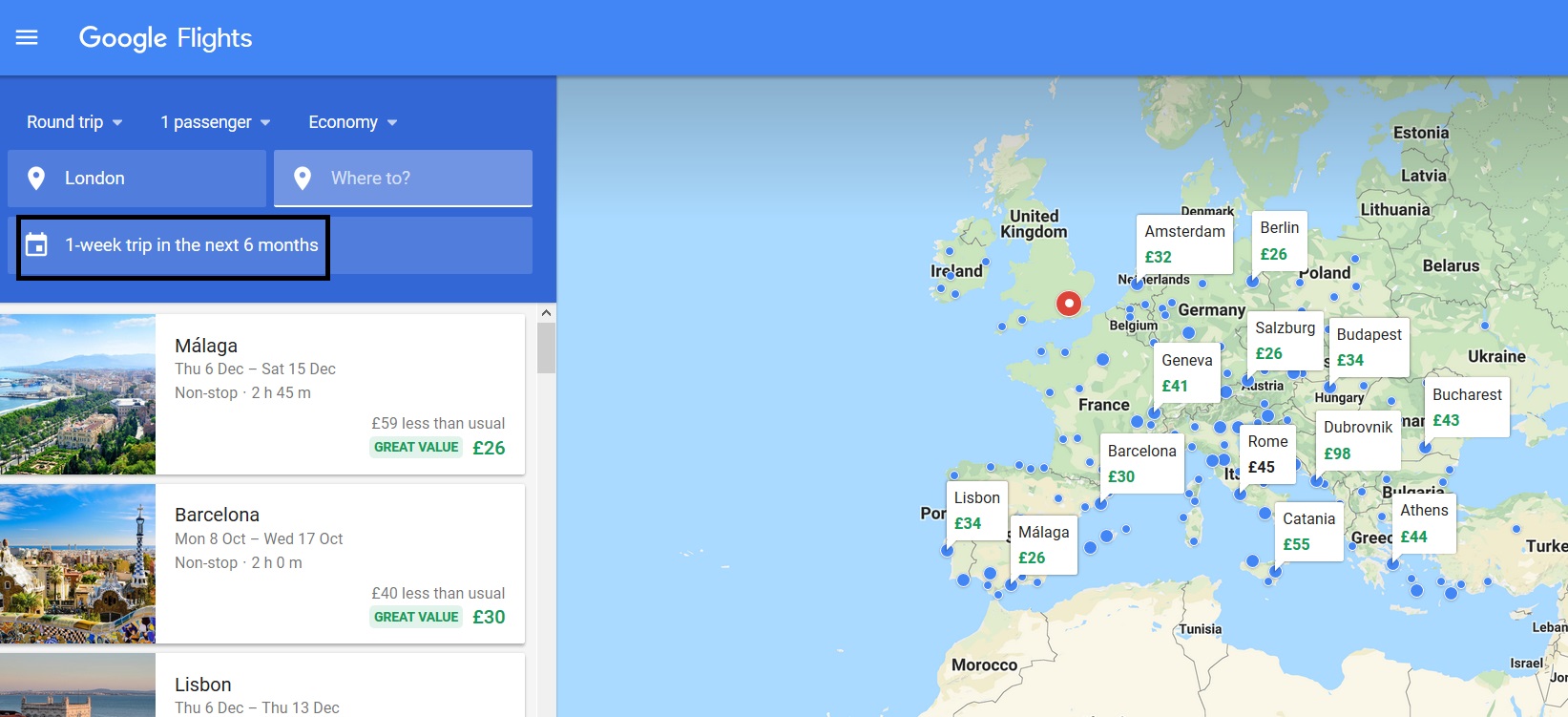This image captures an active session on the Google Flights website. At the top, there is a long, slender rectangle in a deep periwinkle color. On the far left of this bar, three horizontal lines are prominently displayed, followed by the phrase "Google Flights" in white lettering. Below this, a secondary periwinkle rectangle, shorter in length, provides crucial travel details: "Round trip, one passenger, economy." A highlighted bullet point marks the destination as London, and adjacent to it, the text prompts, "Where to?" 

A black rectangular frame encases a calendar interface that specifies, "One week trip in the next six months." Directly beneath this are three labeled boxes indicating popular travel destinations: Málaga, Barcelona (noted as "Barcedona" in the original speech), and Lisbon. The right side of the screen is dominated by a detailed map of Europe, with a marked bullet point highlighting London.